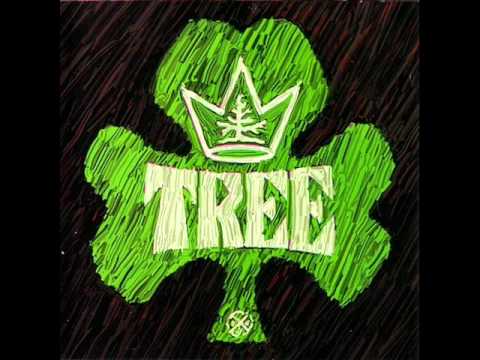The image is a detailed graphic design featuring a vividly textured, green tree set against a black background with intricately aligned, diagonal stripes in brown, gray, and light red accents. The tree is composed of various shades of green lines, giving it a rich, multi-toned appearance. Centered on the tree is the word "tree" written in white with green stripes, adding to the textured, streaky quality. Above this word sits a prominent, three-pointed crown, also in white, with a smaller depiction of a tree in the middle spike. At the base of the tree's trunk, there is a cross within a circle, reminiscent of a railroad crossing sign, adding an additional layer of symbolism to the design.